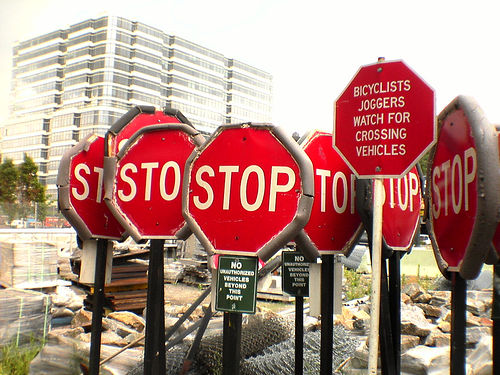The image captures an eclectic array of seven stop signs, most of which bear the classic octagonal shape and vibrant red color with "STOP" inscribed in bold, white uppercase letters. The signs are precariously clustered, with some overlapping others, contributing to a chaotic yet intriguing visual. Two of the stop signs have additional smaller black signs below them stating, "No unauthorized vehicles beyond this point." Additionally, there's one sign that reads, "Bicyclists, joggers, watch for crossing vehicles." These signs exhibit various stages of wear and tear, including rusted edges and faded, chipped paint, indicating they have seen considerable use. The scene is set against an urban backdrop featuring a modern, multi-story building with reflective glass windows. The setting appears to be a construction area, evidenced by scattered wood, rocks, and fencing debris in the foreground. The sky is a pale white, adding to the overall starkness of the composition.